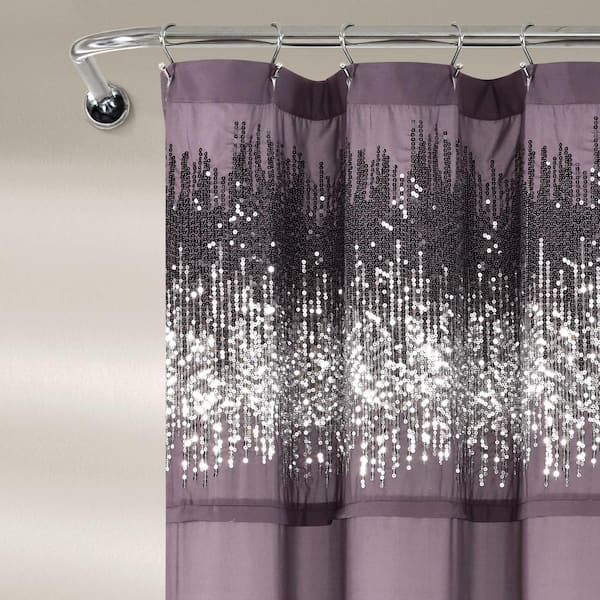The image showcases a close-up of a shower setup featuring a shiny silver shower rod and matching open-ended silver hooks. The focal point is a predominantly purple shower curtain adorned with a pattern of sparkling sequins that form a stripe across the top. These sequins, in both silver and deeper gray, catch the light brilliantly, adding a touch of glamour to the space. The curtain itself features a mix of metallic silver, gray designs, and solid purple sections. The background features a plain, white bathroom wall, with emphasis on the radiant, luxurious look of the curtain and its shiny embellishments.